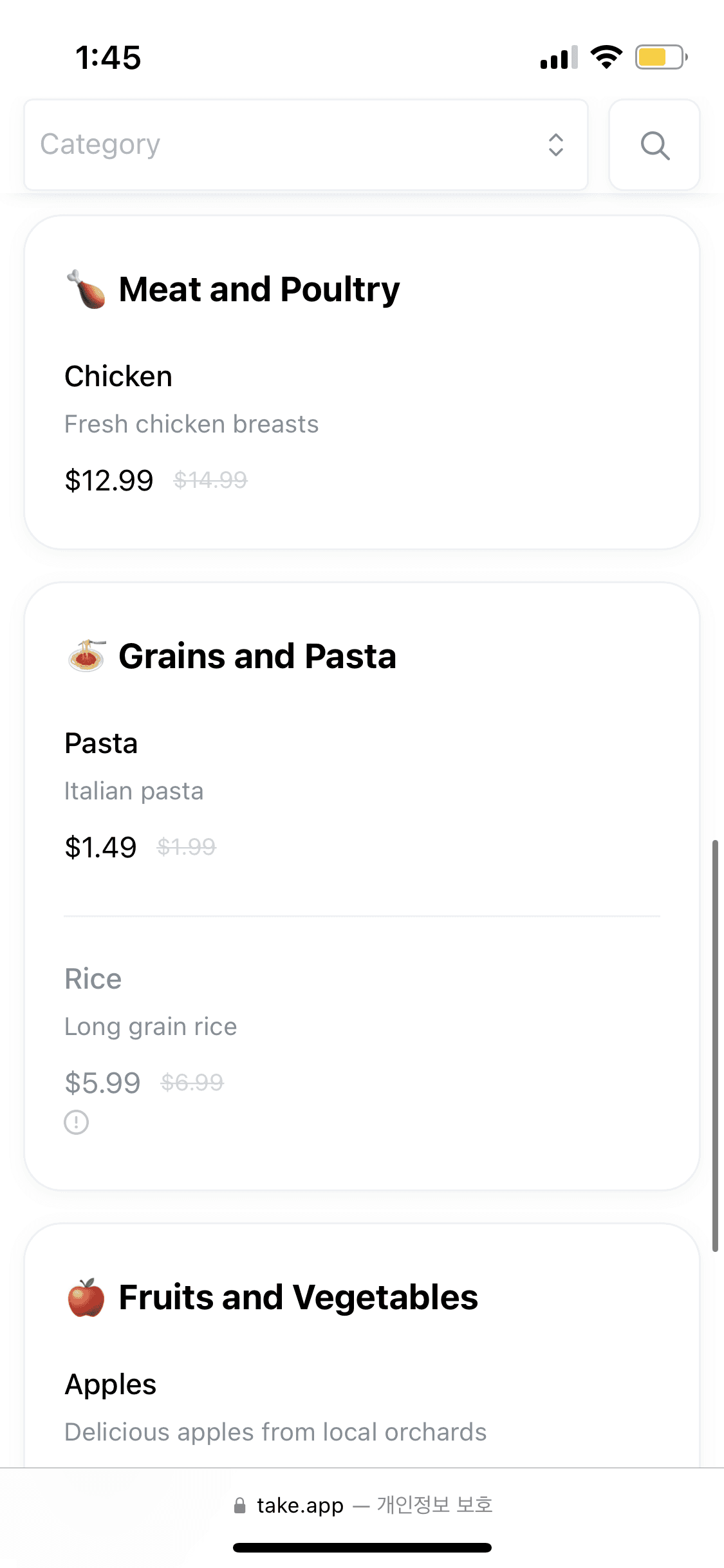A detailed screenshot from someone's iPhone display features a grocery app interface while in a grocery cart. The screen is divided into sections for various food categories. 

In the "Meat and Poultry" section, a cartoon image of a chicken is displayed alongside the text "Chicken, Fresh Chicken Breast." The price is marked at $12.99, reduced from a regular price of $14.99.

Next, in the "Grains and Pasta" section, "Italian Pasta" is listed at $1.49, reflecting a discount from its initial price of $1.99.

The "Rice" section shows "Long Grain Rice" priced at $5.99, with no discount currently applied.

The "Fruits and Vegetables" section mentions "Delicious Apples from Local Orchards," but the price is not visible. The screen indicates further items can be viewed by scrolling down.

At the bottom of the screen, there is a logo and text for "take.app," accompanied by some Japanese or Chinese characters.